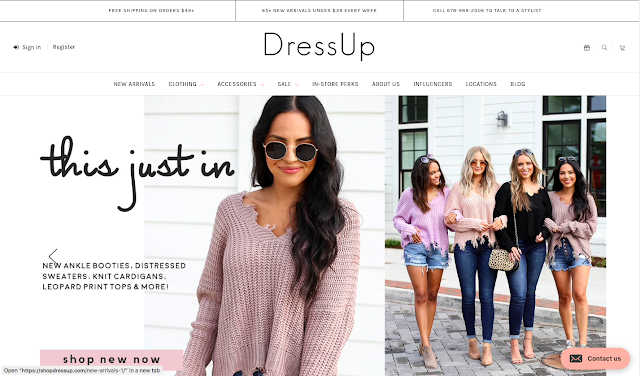**Descriptive Website Screenshot Caption:**

The screenshot showcases a sleek fashion website with a predominantly white background accented by dusky pink elements. At the very top of the site, a minimalist header features two parallel thin gray lines intersected by two vertical lines, creating a button-like element at the center. This header contains three segments of text: on the left, "Free shipping on orders over [unable to read amount]"; in the center, a mention about "New Arrivals"; and on the right, a phone number.

Below this header, the site is center-justified with a clean, modern font reading "DRESS UP", where "DRESS" is in all capitals and "up" starts with a capital "U". In the top left corner of this section, there are "Sign In" and "Register" links. On the right, a search option and two additional icons are visible.

The main navigation bar includes links to "New Arrivals," "Clothing," "Accessories," "Sale," "In-Store Perks," "About Us," "Influences," "Locations," and "Blog".

In the main section of the page, the left side features a brunette model sporting round dark sunglasses and a dusky pink jersey-knit top, set against a white background. To the left of her image, handwritten text reads, "This just in." Below this, promotional text lists "New ankle booties, distressed sweaters, knit cardigans, leopard print tops, and more," accompanied by a left-pointing arrow. Beneath this text is a dusky pink button labeled "Shop New Now."

The right side of the main section displays a vibrant, full-color photo of four women. Two women wear denim shorts while the other two wear denim jeans, all adorned in various styles of cardigan tops. From left to right, their cardigans are a bright pinky-mauve, pale pink, black, and dusky pink. They stand on a cobblestone street in front of a white building with large windows. In the bottom right corner of the page, another dusky pink button reads "Contact Us," featuring an envelope icon.